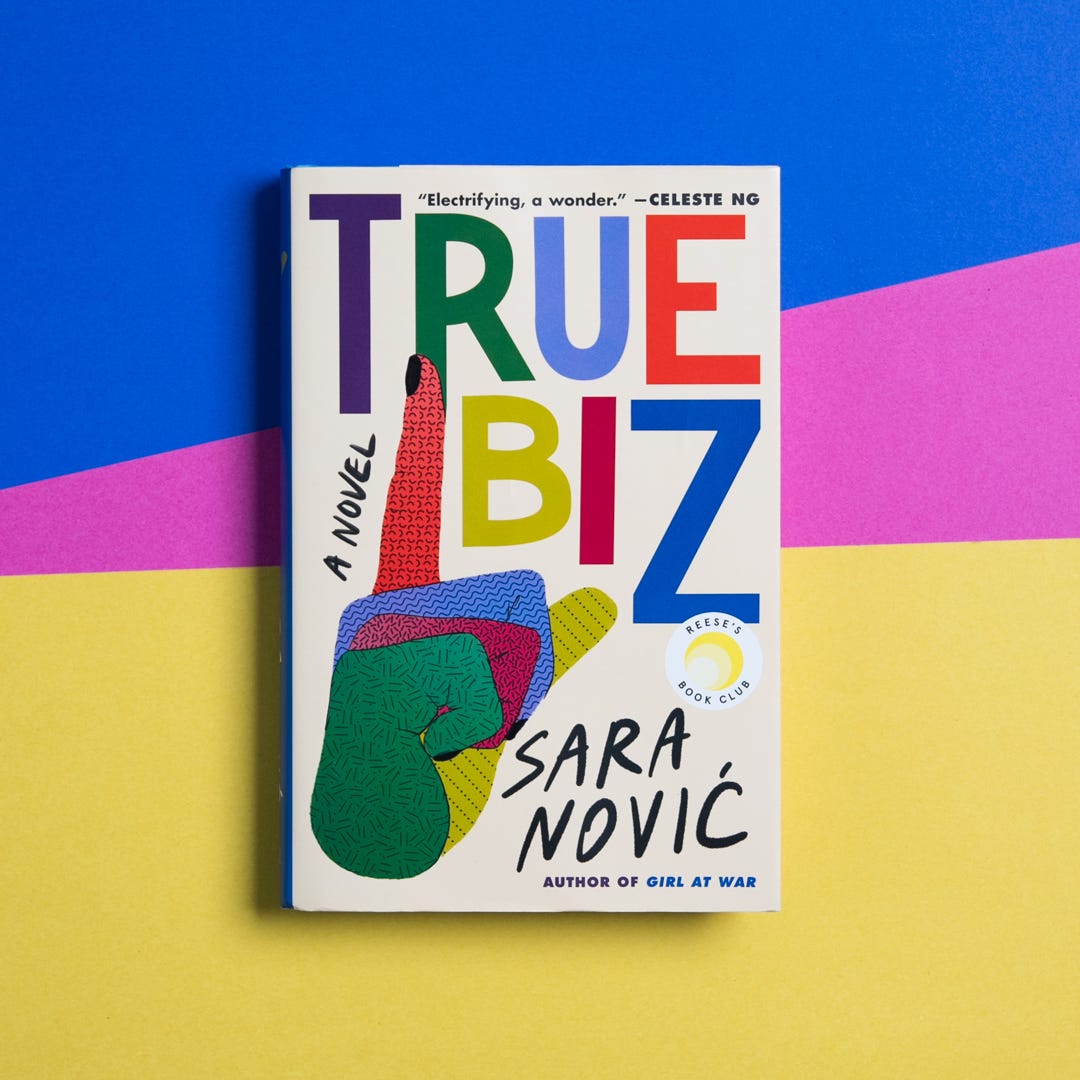The image depicts the cover of the book "True Biz" by Sarah Nović, set against an abstract background transitioning from yellow at the bottom, through purple in the middle, to blue at the top. The yellow section, the largest and nearly rectangular with a slight positive slope, separates from the triangular purple section, which itself transitions to a right triangle of blue, marked by a clipped apex on the right edge. The title "True Biz" is written in vibrant, multicolored letters: T (purple), R (green), U (blue), E (red), B (yellow), I (reddish-purple), and Z (dark blue). A commanding human hand, adorned in a multicolored, glove-like design, showcases its index finger pointing upwards with black nail polish, blue-curled middle finger, purple ring finger, green pinky finger, and yellow thumb resting on the second finger. Above the hand is the acclaim: "A novel, electrifying, a wonder," by Celeste Ng. The author, Sarah Nović, known for "Girl at War," has her name noted at the bottom of the cover. The comprehensive scene and vibrant hues create a striking visual appeal.